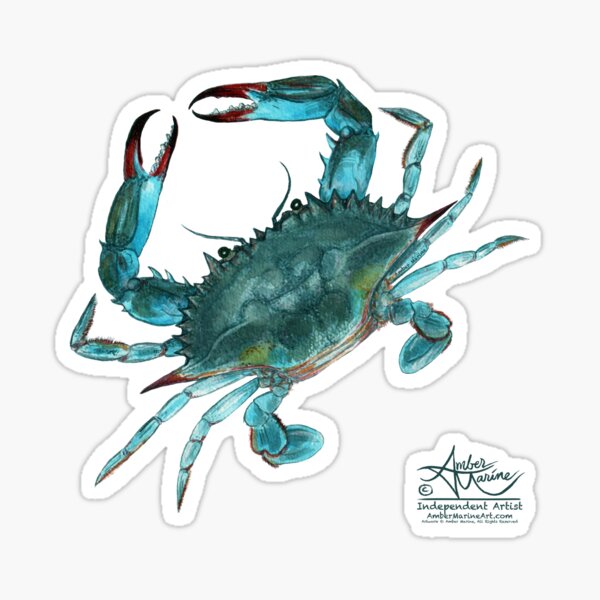This is an image of a sticker featuring a detailed illustration of a blue crab, primarily depicted in various shades of blue and teal. The tips of the crab's claws are highlighted with shades of red and maroon, adding a striking contrast to its predominantly blue exoskeleton. The crab's body also contains some subtle hints of green and teal. With a watercolor-like artistic style, the crab is oriented with its claws and eyes facing the upper left corner, while its rear legs point towards the lower right. The sticker itself has an opaque, solid white background, bordered by a light grey outline. At the bottom of the sticker, the text reads "Amber Marine" in stylized dark ink script, followed by "Independent Artist" in smaller font below. There is also a partially legible URL, "ambermarineart.com," but the finer details are too small to read clearly.